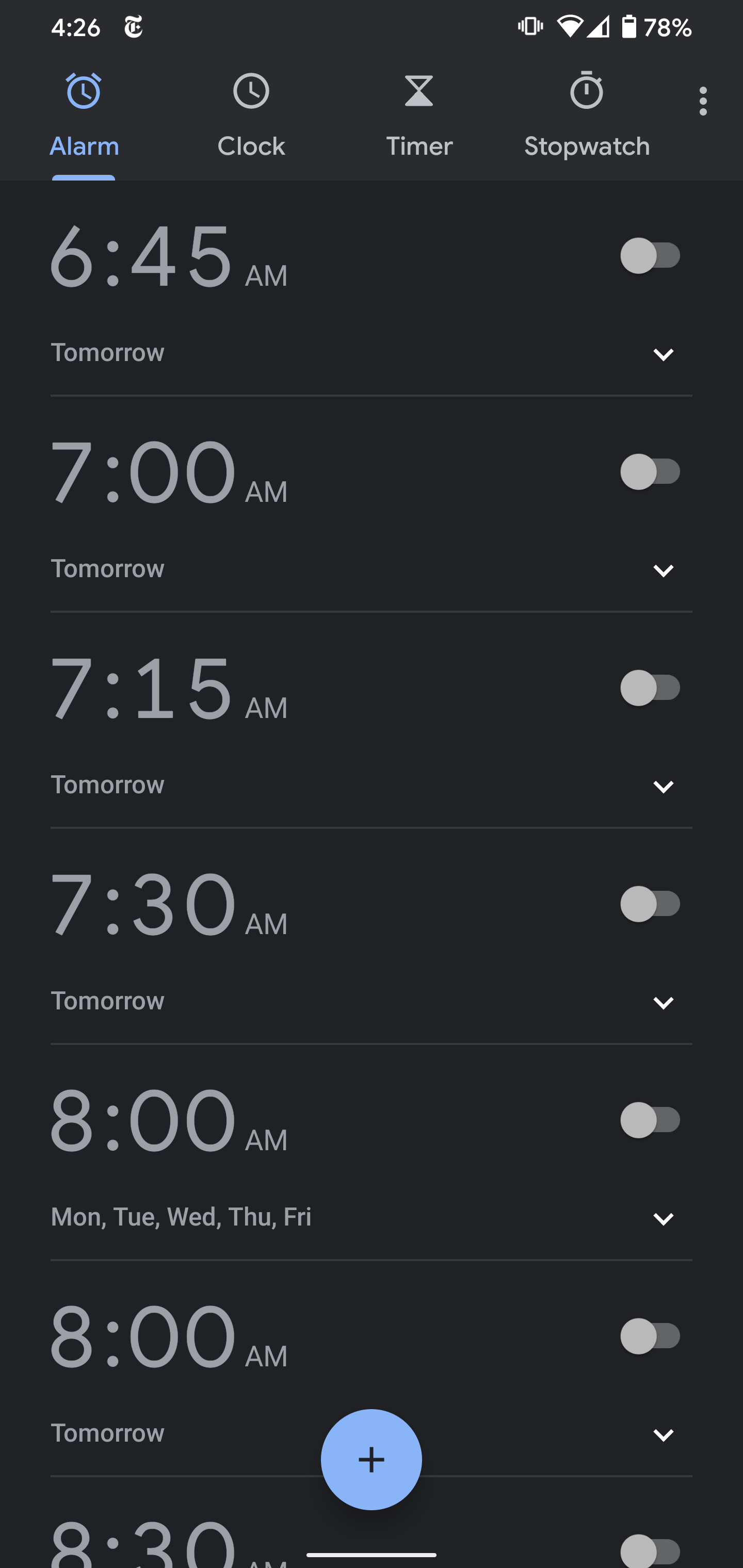This screenshot captures the alarm settings section of a cell phone. The background is predominantly black. In the top left corner, the small white text displays the current time as 4:26. Adjacent to this is a New York Times icon, indicating that the New York Times app is open. The very top section of the screenshot showcases various status icons from left to right: vibrating phone, Wi-Fi, phone signal strength, battery level indicator, and the battery percentage in the top right.

Beneath these indicators, four horizontally aligned icons represent different functions: Alarm, Clock, Timer, and Stopwatch. The 'Alarm' icon is currently selected, highlighted in light blue with a corresponding light blue line underneath it.

Following this, a vertical list of pre-set alarm times is displayed, with each time shown in large gray numbers on the left. Adjacent to each listed time is a toggle switch, which allows the user to easily turn individual alarms on or off.

At the bottom center of the screen, a prominent blue circle with a plus icon invites the user to add a new alarm. The overall layout is intuitive, making alarm management straightforward and accessible.